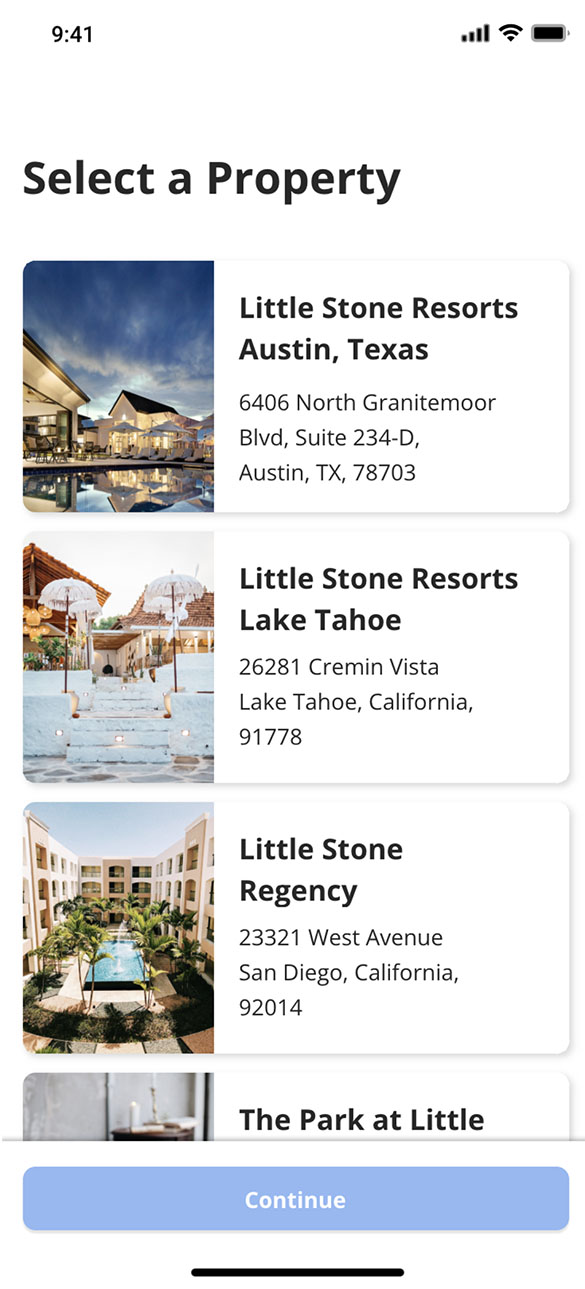This image is a screenshot of a resort and hotel booking application displayed in a rectangular format. The vertical sides of the image are longer than the horizontal sides. The entire background is white, providing a clean and simple interface. Each listing within the application is presented in its own segmented rectangular box. These boxes feature a photo occupying the left third, and the right two-thirds contain resort information on a white background with black text. 

Each listing is separated by a thin white line, and the rectangles have a light gray shadow effect applied, which creates a subtle 3D appearance, adding depth and dynamism to the design. At the bottom of the image, a white banner holds a blue, rectangular button marked with white text that reads "Continue," indicating it is an interactive element for user progress.

At the top of the image, in black text, it states "Select a property" on a white background, initiating the selection process. The first listing showcases a tan-colored resort featuring multiple umbrellas and beach chairs next to a pool. To the right, the black text reads: "Little Stone Resorts, Austin, Texas, 6406 North Granite Moor Boulevard, Suite 234-D, Austin, Texas, 78703."